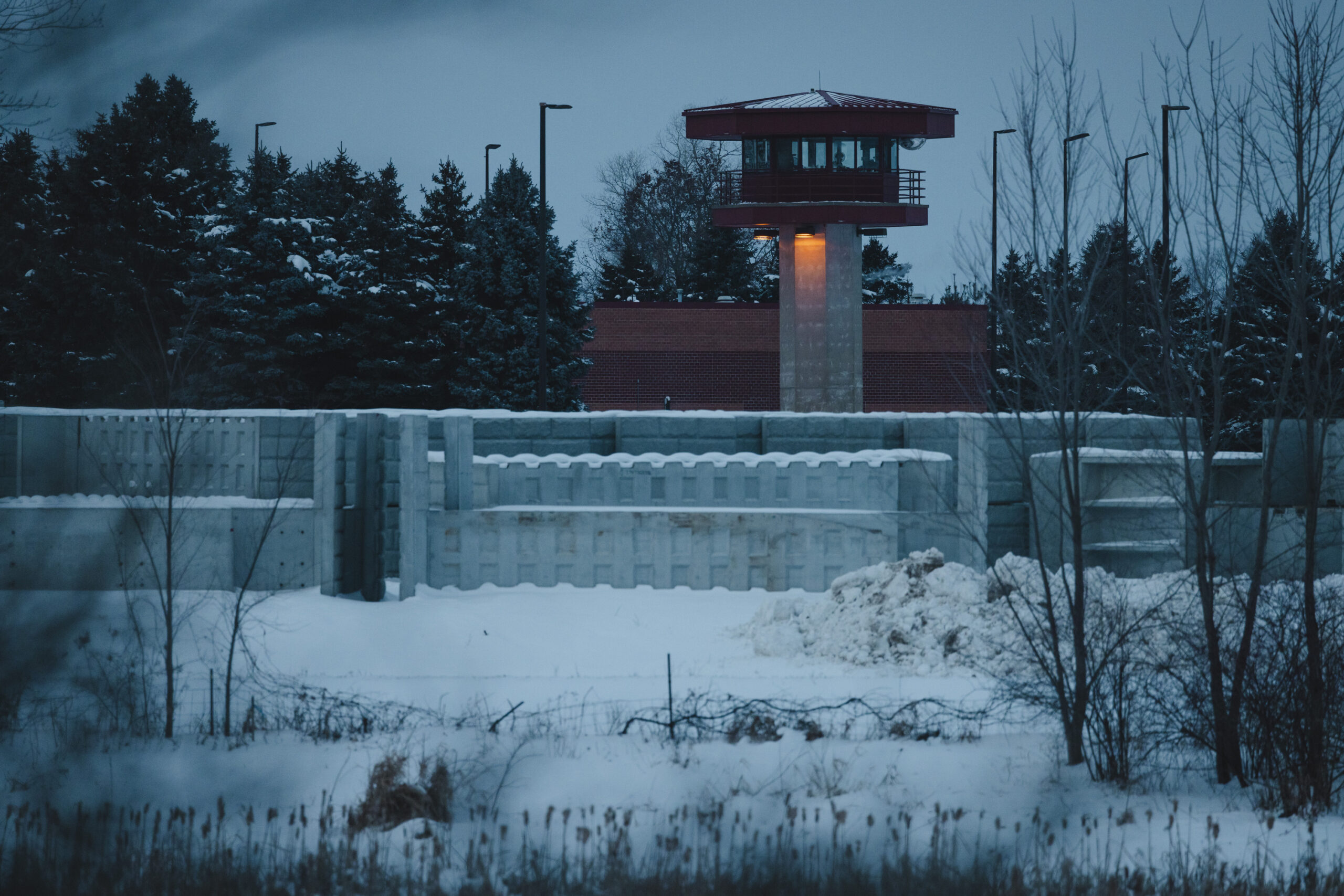The photograph captures a snowy, low-light scene of a prison yard in winter, with a sense of desolation and containment. The foreground features dormant, yellowed grass and what appear to be cattails along a creek, all blanketed in thick, white snow. In the middle ground, bare, leafless trees stand starkly against the snowy landscape, interspersed with piles of snow. The prison yard is encircled by a high concrete wall, topped with barbed wire for added security. Dominating the scene is a round guard tower on a concrete pedestal, its snow-covered roof and illuminating lights casting a glow below. The tower, equipped with windows and an exterior circular walkway, is positioned well above the surrounding wall, providing a vantage point for surveillance. Beyond the yard, tall conifer trees—likely fir or pine—form a dense line, their branches also heavy with snow. The low brick prison building with a brown roof is visible, and tall security lights on poles loom like sentinels throughout the yard. The sky, painted a gray-blue hue, hints at the fading light of late afternoon, enhancing the cold and isolated atmosphere of the scene.